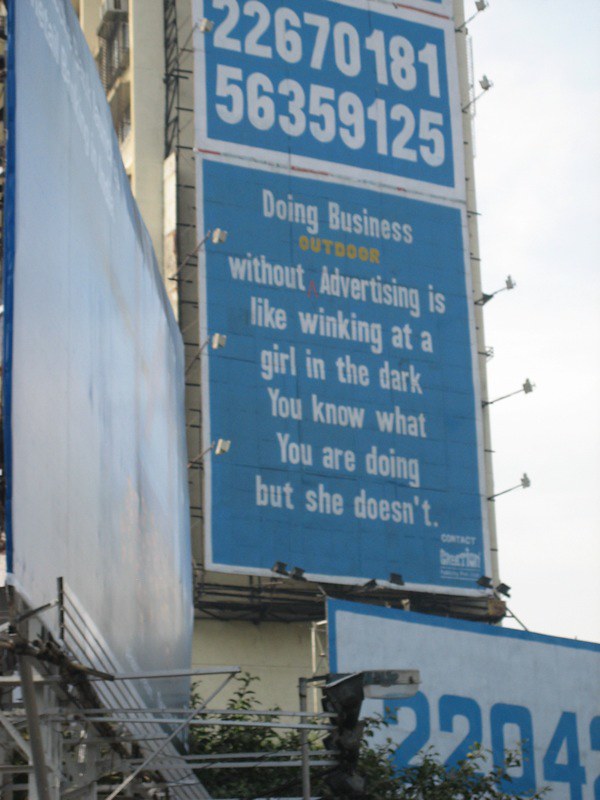In this vertical daytime photograph, three billboards are prominently displayed against a backdrop of an overcast, white sky. The lower left of the image features a blank billboard, accessible via silver metal stairs. Centered above this, a second billboard dominates with text descending from the top of the frame. It reads: "Doing business without advertising is like winking at a girl in the dark. You know what you are doing, but she doesn't." In the lower right corner, a third billboard with a white background and blue border showcases a large blue number: "2204." The image captures a scene of urban advertising infrastructure, highlighting both the potential and the necessity of visible messaging.